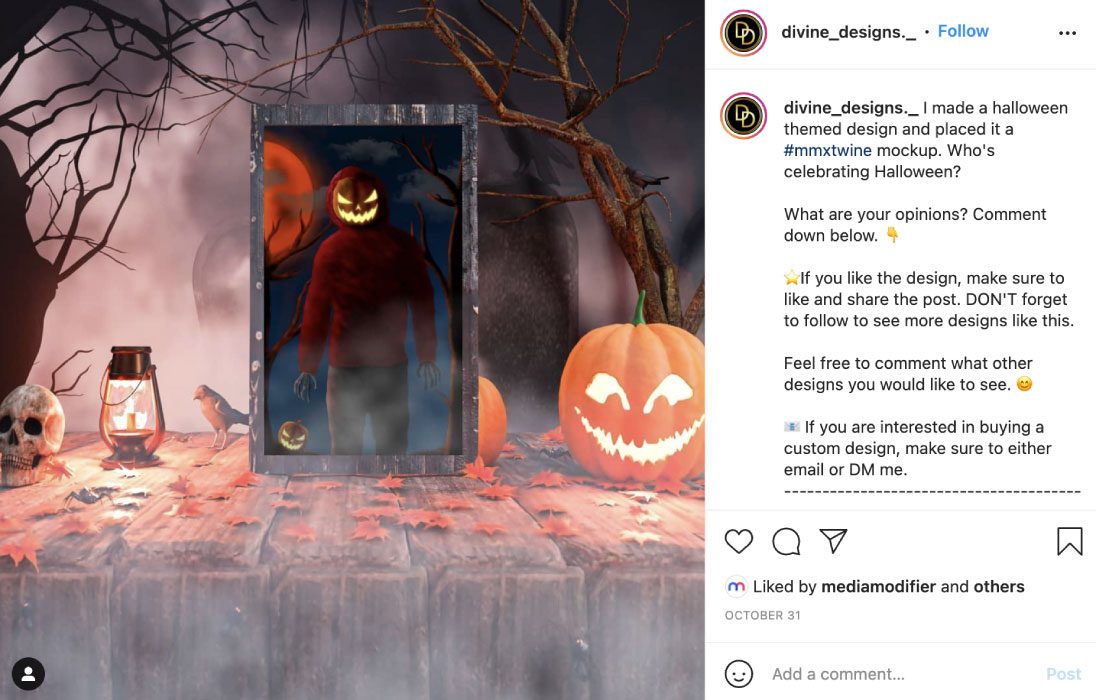This is a screenshot of an Instagram post from the user account Divine Designs, featuring a meticulously crafted Halloween-themed photograph. The backdrop of the image is a misty, gray sky, hinting at an eerie cemetery scene where the vague outlines of tombstones materialize through the dense fog. Flanking the central figure are two gnarled, lifeless trees, amplifying the spooky ambiance.

At the heart of the photo stands a haunting figure clad in a long-sleeved red shirt, adorned with skeletal hands and a terrifying mask. The figure ominously cradles a luminescent jack-o'-lantern, casting a ghostly glow. This person is positioned within a ornate dark gray mirror, which acts as a portal to an even more haunting dimension. Within the mirror's reflection, the figure is again framed by two barren trees, and a menacing dark orange moon looms large in the background.

Surrounding the mirror, an assortment of macabre decorations rests upon a weathered wooden surface with vertical planks. The items include a pitch-black crow, a vintage oil lantern, a sinister skull, additional glowing jack-o'-lanterns, and scattered dead leaves, further enhancing the Halloween spookiness. An icon of a person is discreetly placed in the bottom left corner, indicating the social media nature of the post.